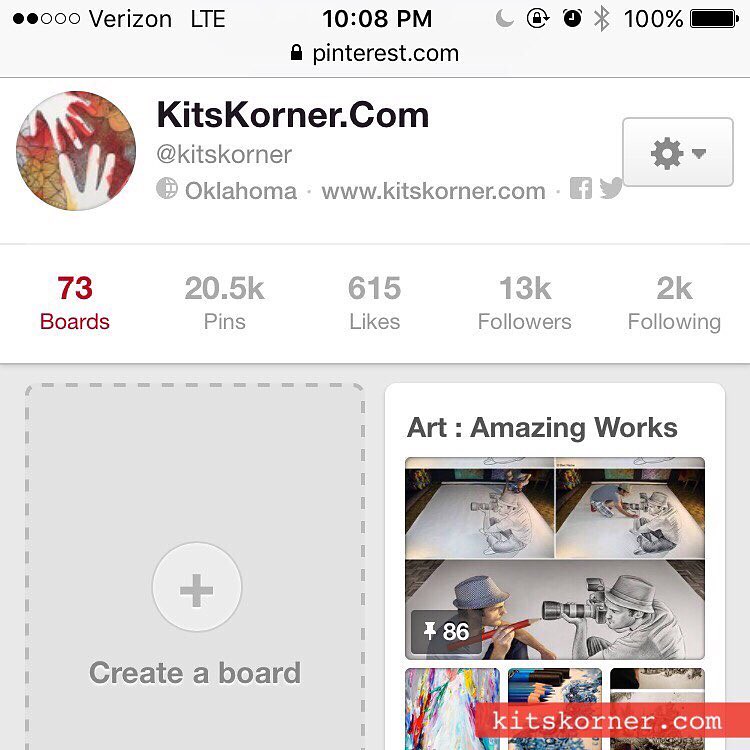The image is a detailed screenshot from an iPhone using the iOS operating system, displaying a Pinterest profile page for KitsCorner.com. The screenshot features a light gray header bar indicating it's 10:08 PM, the device is connected to Verizon LTE, and the battery is fully charged at 100%. The header includes icons for a half moon, a lock with a circular arrow, a clock, and Bluetooth status.

Beneath this, the main content area presents the KitsCorner Pinterest profile. The profile's avatar is a circle displaying a watercolor painting with white hands over orange and red patches. To the right of the avatar, bold black text reads "KitsCorner.com," followed by the username "@KitsCorner," indicating its location in Oklahoma, along with the website URL and icons for Facebook and Twitter.

The profile statistics reveal 73 boards, 20.5K pins, 615 likes, 13K followers, and 2K following. The screen is divided into two main sections below the profile information. On the left, a darker gray area features a circle with a plus sign, labeled "Create a Board." On the right, against a white background, there is a section titled "Art: Amazing Works," showcasing 86 pinned artworks. Among these, one prominent piece appears to be a step-by-step illustration of a perspective drawing that gives an illusion of popping out of the page. The capture elaborates the colorful palette throughout, depicting black, white, red, green, purple, yellow, and orange hues.